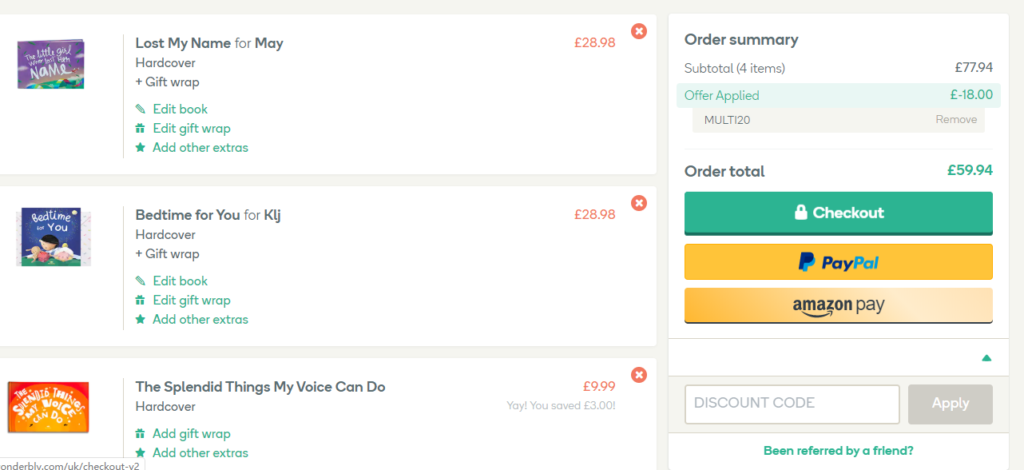This is a detailed screenshot of a checkout screen on a website. On the left side, there are three items listed, each presented on a white rectangular background and separated by thin gray lines. 

1. The first product listed is "Lost My Name for May," which includes a hardcover book and gift wrap. Beneath this, there are options in green text: "edit book," "edit gift wrap," and "add other extras." The price for this item is displayed in orange text as £28.98, with an orange circle containing a white X in the top right corner for removal.

2. The second product is "Bedtime For You for KLJ," also a hardcover book with gift wrap. Similar editing and additional options are listed: "edit book," "edit gift wrap," and "add other extras." The price is again £28.98 in orange text, with an orange circle with a white X for deletion.

3. The third item is "The Splendid Things My Voice Can Do," a hardcover book that includes options to "add gift wrap" and "add other extras," though its bottom is cut off in the screenshot. The price for this item is £9.99, which is followed by a light gray text stating, "yay, you saved £3!"

On the right-hand side is the checkout information, presented on a white background:

- The order summary begins with the subtitle, "4 items," showing a total of £77.94. 
- A discount is applied, visible in a green box with "minus £18."
- Below this discount, a gray box displays the text "Multi 20," with light gray text to the right stating "remove."
- Finally, the "order total" is shown in teal as £59.94.